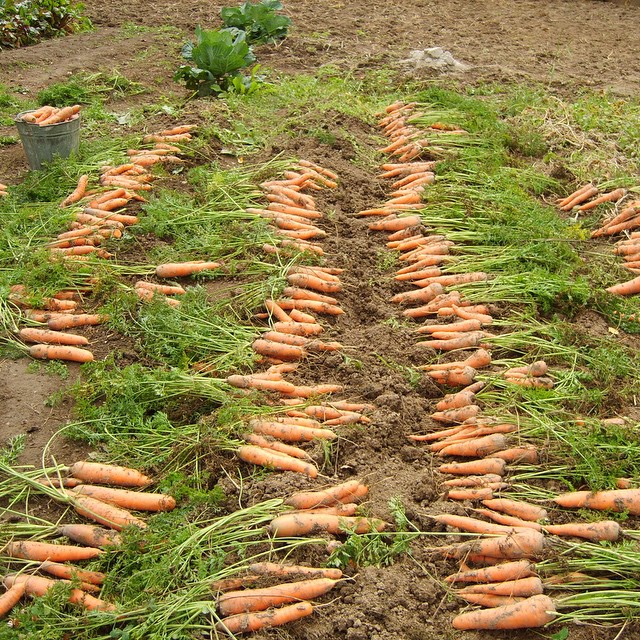The image captures a vibrant scene of a freshly harvested carrot field during the daytime. Rows of carrots, numbering in the hundreds, stretch horizontally across the brown soil. Each carrot lies neatly with its green stems still attached, varying in size and shades of orange, some still dusted with the earth from which they were pulled. To the left of the rows sits a grayish, metal bucket brimming with more harvested carrots. Beyond the carrot rows, there are two leafy heads of lettuce, and to the far right, an expanse of tilled soil lies ready for planting. The entire scene is accentuated by the natural, rustic setting of the garden or field, emphasizing the bounty of the harvest.